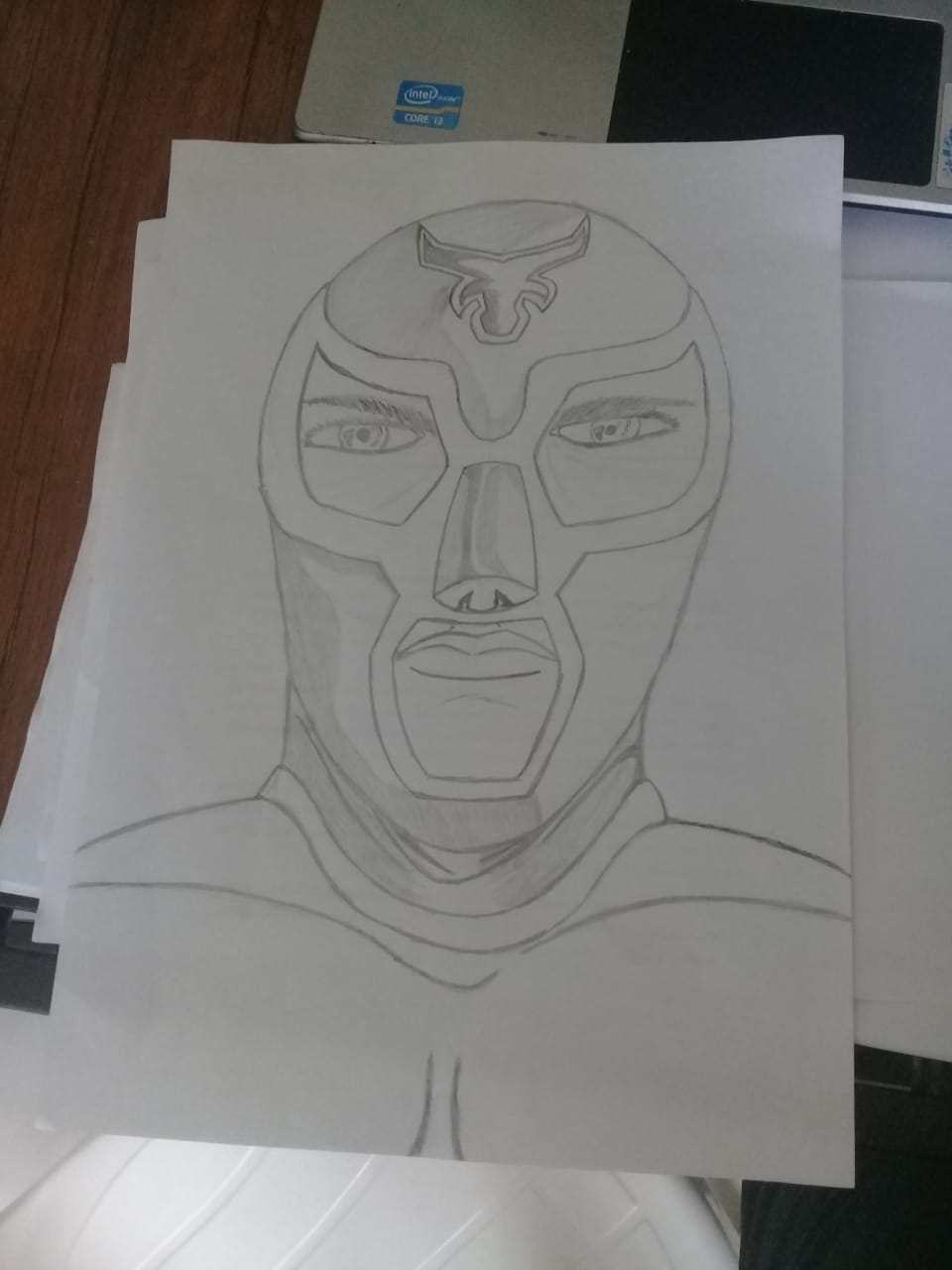The image is a detailed pencil drawing presented in black and white, depicting a figure that appears to be either a superhero or a wrestler. The character is adorned with a distinctive mask featuring a ram or bull-like symbol emblazoned on the forehead. This mask covers the area around his eyes, extends over his cheeks, and wraps around his neck, where faint wrinkles are visible. The mask also allows a view of the man's eyes, eyebrows, mouth, and nose, with a cutout specifically highlighting his lips. His upper body is muscular, suggested by the outlines of his pectoral and trapezoid muscles, with what looks like a cape draped from his shoulders. The drawing lies atop several other sheets of white paper, all situated on a wooden table. In the background, there's an additional piece of paper or cardboard with two blue cutouts. At the top right of the image, a laptop with a visible touchpad can be seen, and below all of this, a white plastic chair is also visible.